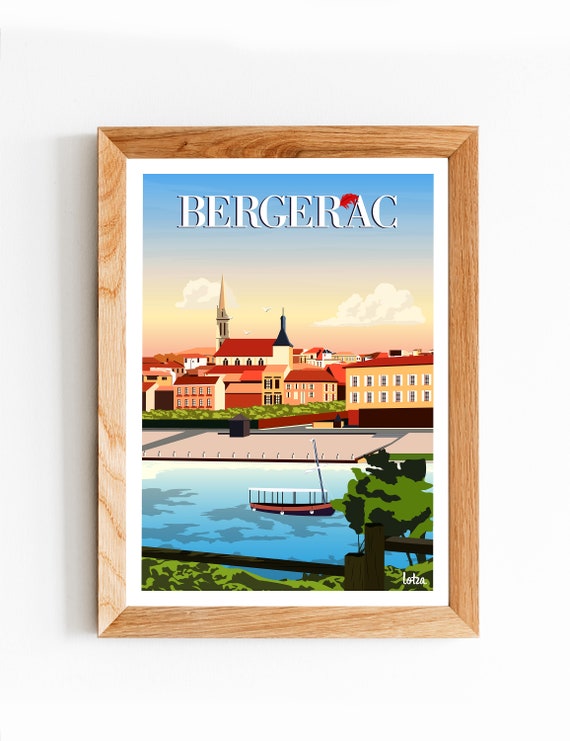The framed photo features a picturesque landscape, enclosed in a wooden frame. The sky within the frame transitions from a deep blue at the top to a soft, golden yellow near the horizon, dotted with scattered white clouds. At the base of the image, a lush green tree is prominently depicted, providing a natural contrast to the serene blue body of water below, which appears smooth and glossy. In the background, there are several buildings with striking ruby red rooftops, their rich color adding a vibrant touch to the overall scene.